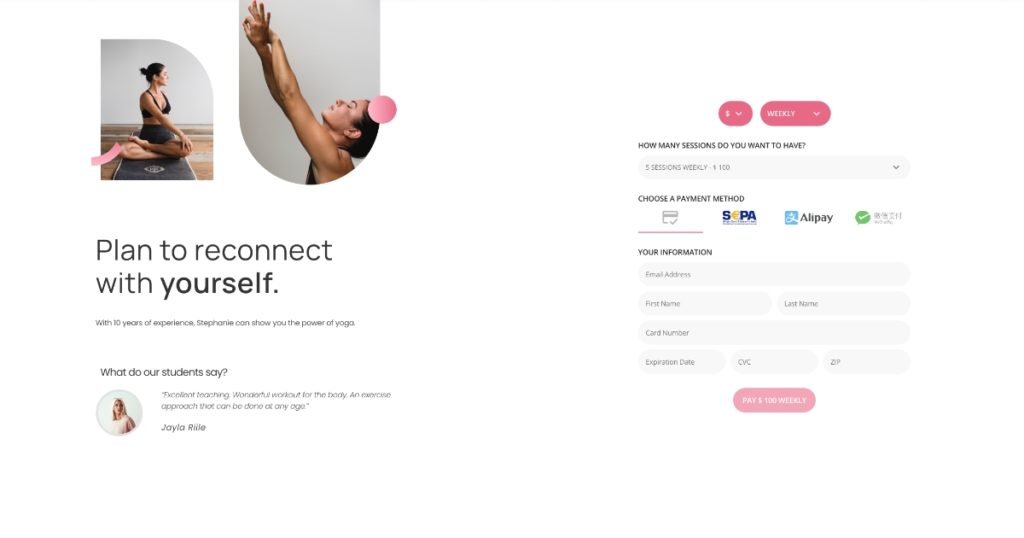Here is a detailed and cleaned-up caption for the image described:

The image is a screenshot of what appears to be a promotional interface for a yoga class. At the top left, it showcases two images of a woman practicing yoga. In the first image, she is seated in a cross-legged position, looking off to the side with her upper body turned away from the camera. In the second image, she is stretching her arms upwards and has her eyes closed, conveying a sense of tranquility. Below these images is the text, "Plan to reconnect with yourself." Further down, smaller, unreadable text is present, followed by larger text saying, "What do our students say?" 

Accompanying this is a testimonial from a woman, presumably named Jayla, whose picture is attached to her quote. On the right side of the image, there are two drop-down menus for selecting the number of sessions and the frequency of participation, with the options currently set to six sessions weekly. Beneath these selections is a question, "How many sessions do you want to have?" accompanied by a blank drop-down box. Below this is the payment section with the text "Choose a payment method," where "Credit Card" is currently selected. Other options include "S Pay" and "All Pay," next to a green check mark whose function is unclear. Further down, there's a section labeled "Your Information" with the usual fields for entering credit card details. At the top right corner, a prominent pink button labeled "Pay Weekly" is displayed.